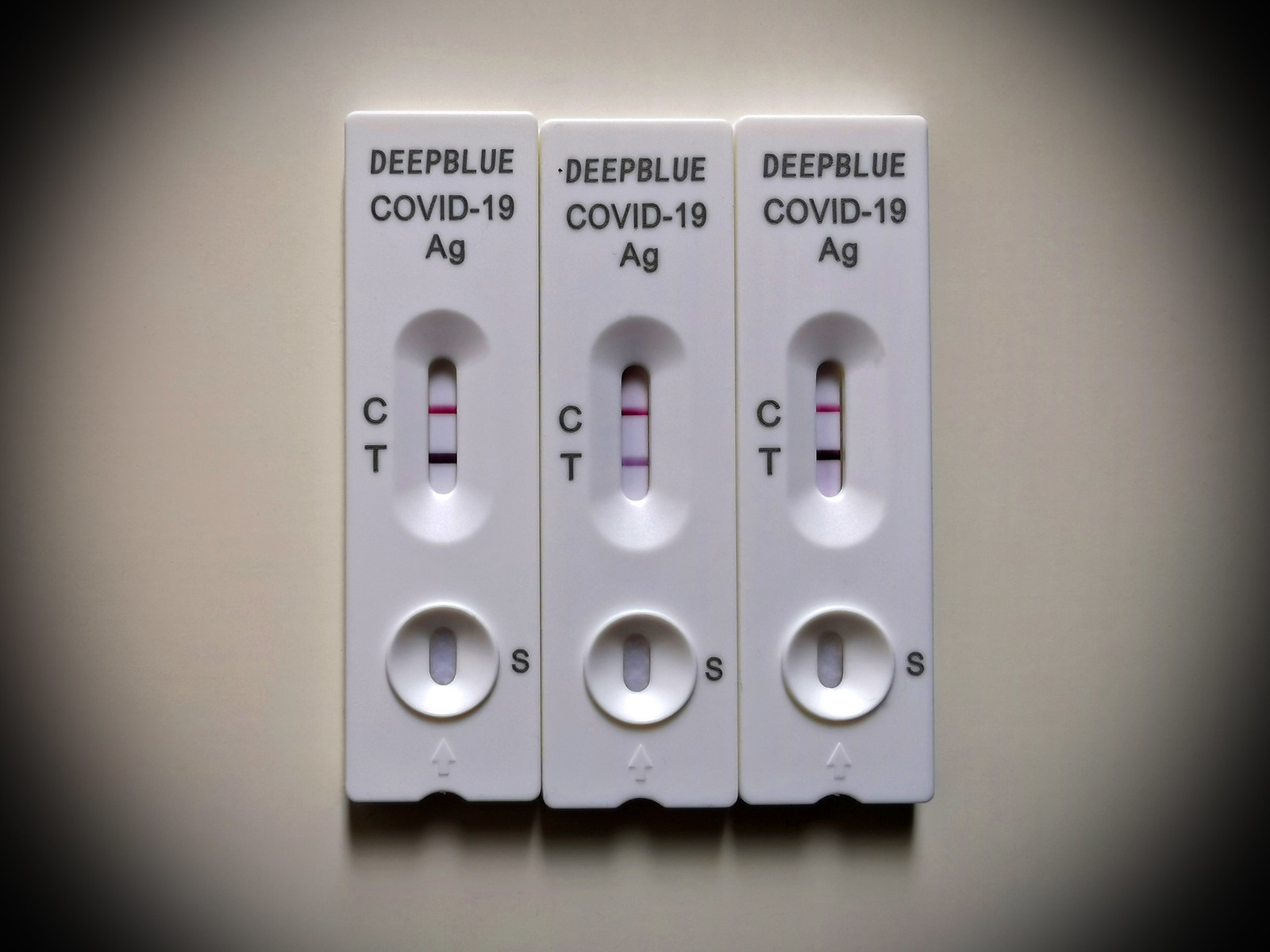The image features a black vignette frame effect at each of the four corners, creating a blur that contrasts against the predominantly white background. Centrally placed within the image are three COVID-19 rapid antigen tests, branded "Deep Blue COVID-19 AG."

Each test displays a control (C) and test (T) line printed in stark black. All three tests show a dark maroon red line at the control (C) position. Likewise, the test (T) positions on the outer two tests exhibit thick black-red lines, indicating a positive result. The middle test, however, has a test line (T) that is a faint purple, which still suggests a positive result albeit less pronounced.

At the bottom section of the tests, there is an 'S' with a circle adjacent to it, and an arrow pointing towards the circle. Inside the circle is an oblong shape that bears a passing resemblance to a pill, symbolizing the sample application area.

These tests lie used and indicate positive results, suggesting that they were taken by either a single individual consecutively or by multiple individuals, possibly in a family setting or at a healthcare facility.